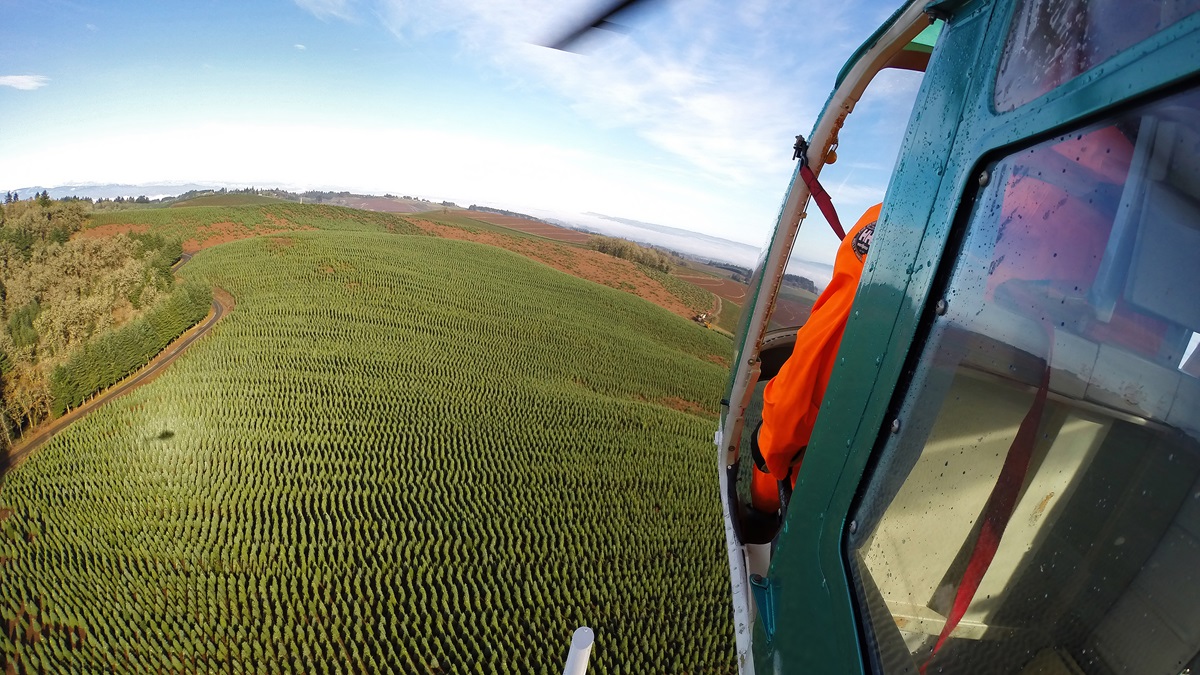The image is an overhead, slightly angled view taken from a helicopter, with the camera positioned on the side of the aircraft. The helicopter is painted in a greenish-aqua hue, and a small shadow of the helicopter can be seen below, confirming its presence. The left arm of the pilot, dressed in an orange jacket with a patch on the shoulder and the door wide open, is visible. Additionally, a tiny bit of one of the helicopter blades can be seen at the top edge of the frame. The expansive field below is lush and green, with some areas showing the potential of crops growing in somewhat curved rows. To the left, some trees break the uniformity of the greenery. The scene conveys a sense of isolation with no visible roads, people, or animals. The sky above is light blue with white clouds, adding to the daytime atmosphere. The horizon is flat and somewhat foggy, suggesting proximity to the sea or expansive flatlands in the distance.